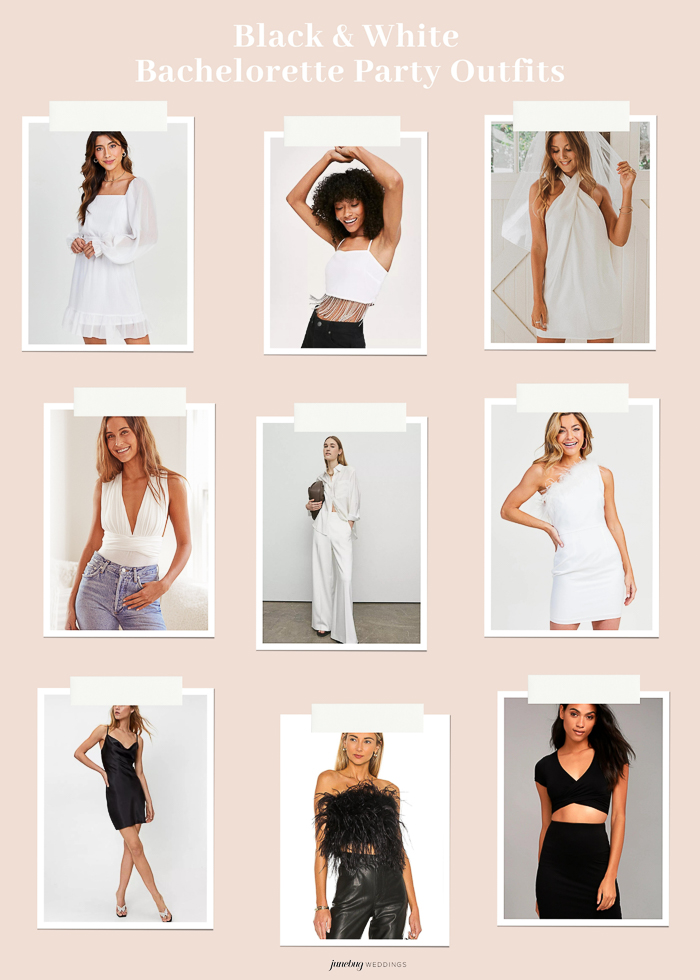The image features a rectangular collage, measuring approximately 6 inches high by 3 inches wide, with a light dusty pink background. At the top, white text reads, "Black and White Bachelorette Party Outfits." There are nine individual pictures organized in a 3x3 grid. Each picture showcases a different woman against a plain backdrop.

- **Top Left:** A woman with long brown hair, wearing a white dress with long sleeves and a necklace.
- **Top Middle:** A woman of African descent with large curly black hair, wearing a fringed crop top and black jeans, raising her arms as if dancing.
- **Top Right:** The apparent bride with long blonde hair, wearing a short white wedding dress with a wrap-around neck and a white veil.
- **Center Left:** A blonde woman with long hair, wearing a white halter top and blue jeans.
- **Center:** A woman with blonde hair in a white button-up shirt and long, loose-fitting white pants.
- **Center Right:** A blonde woman in a white off-shoulder dress with feather details around the neckline.
- **Bottom Left:** A Caucasian woman, partially cropped, with long blonde hair and wearing a low-cut, black silk dress or slip.
- **Bottom Center:** A blonde woman in a feather-covered crop top paired with black leather pants.
- **Bottom Right:** A woman with light brown skin and long dark hair, dressed in a black crop top with sleeves and high-waisted pants.

At the bottom middle of the image, black text reads, "Junebug Weddings."